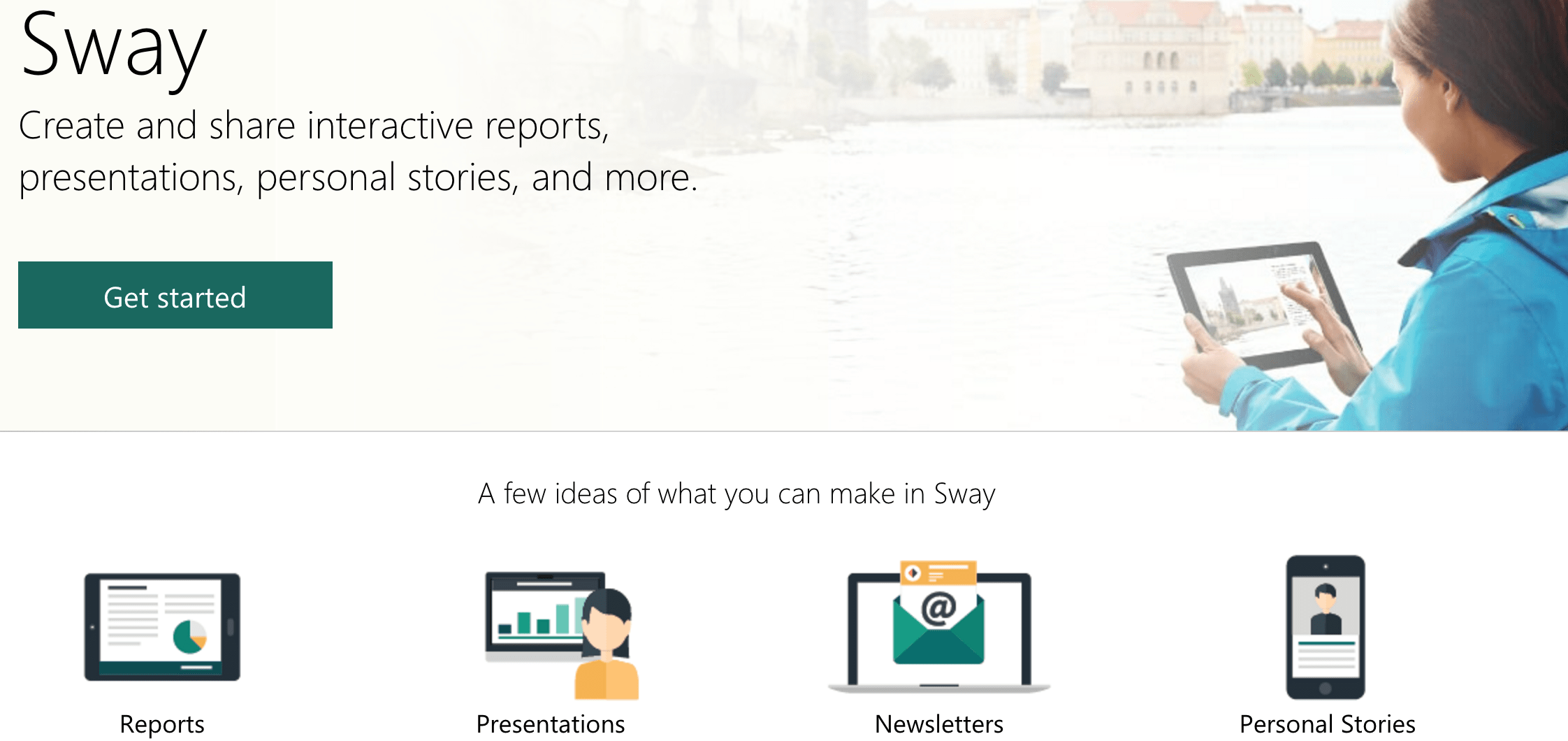The image showcases the homepage of the Sway website, which prominently features the Sway logo rendered in black text with a capital "S" followed by lowercase "w-a-y." Below the logo, a tagline reads: "Create and share interactive reports, presentations, personal stories, and more." A green button labeled "Get Started" is prominently displayed beneath the tagline.

To the right of the text, there is an image of a young girl with long hair, wearing a blue windbreaker jacket. She is holding a tablet horizontally with her left hand, while her right hand is positioned to interact with the screen.

Below this section, a thin gray line extends horizontally from the left to the right side of the image. Beneath this line, centered in the middle of the image, is the text: "We have a few ideas of what you can make in Sway."

Following this text are four categories, each represented by an animated image. The first category, "Reports," is depicted with a corresponding report image. The second category, "Presentations," is illustrated with a presentation board featuring a woman icon. The third category, "Newsletters," is represented by a laptop with an envelope containing a letter and the "@" symbol. The final category, "Personal Stories," is shown with a cell phone displaying an animated man.